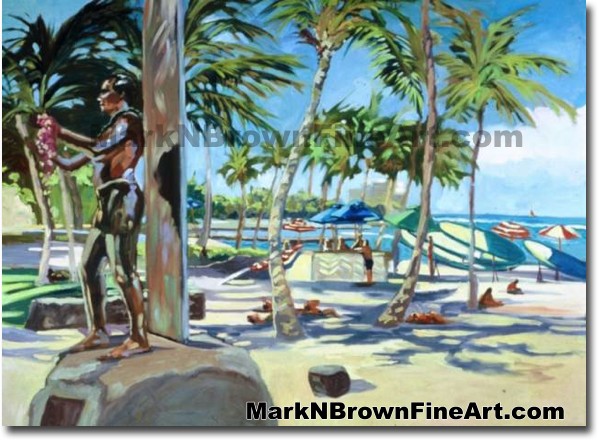The painting depicts a vibrant beach scene, possibly set in Hawaii given the presence of palm trees and a man possibly holding a lei. The sky is a bright turquoise with a few clouds, and the scene is bathed in sunlight, indicating a nice day. Green palm trees with beige trunks frame the backdrop, while the beige-yellow sand stretches across the foreground. There’s an array of blue, red, and white umbrellas dotting the shore, with people seen enjoying the beach—some holding surfboards and others in the water.

In the foreground to the left, a man with dark-colored skin stands on a large rock with a pole behind him, resembling a statue. He is dressed in a bathing suit and gazes to the left, holding something that appears to be a lei, enhancing the tropical vibe. The scene includes patches of green grass and shadows of palm trees, adding depth to the composition.

The artwork is detailed and colorful, capturing the essence of a tropical paradise. The painting is credited at the bottom with the watermark "marknbrownfineart.com" in black font, with the first letters of each word capitalized. This URL appears twice, once as a watermark and once in the bottom-right corner.